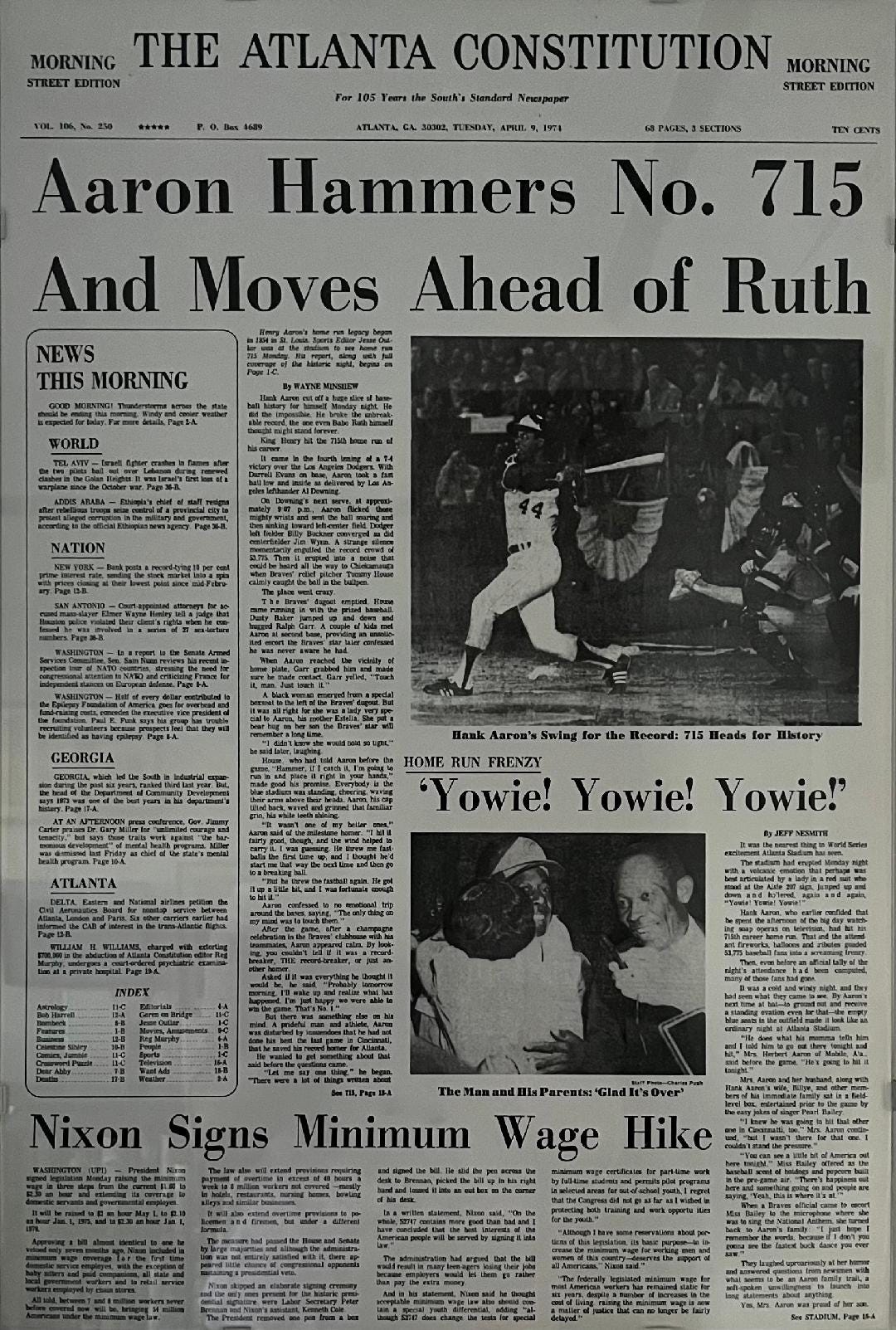The image depicts the front page of an old newspaper titled "The Atlanta Constitution" with a predominantly white background. At the top, in bold black letters, the newspaper name is flanked on either side by the words "Morning Street Edition." Below this header is a subheading in bold that reads: "Aaron hammers number 715 and moves ahead of Ruth." The headline commemorates Hank Aaron's historic achievement of breaking Babe Ruth's all-time home run record. 

To the right under the headline, there is a black and white photograph of Hank Aaron swinging a baseball bat while wearing a white jersey with the number 44 on it. Beneath this main image, a smaller photograph shows Hank Aaron hugging two individuals, likely his parents, with the caption indicating their relief that the pursuit of the record is over. On the left side of the image, text in small black font comprises several unreadable paragraphs forming a news article about Aaron’s milestone.

Adjacent to this article on the left side, a large vertical rectangular box outlined in black is prominently displayed. At the top of the box, the text "News This Morning" appears, followed by headers such as "World," "Nation," "Georgia," and "Atlanta," each underlined with a short paragraph beneath them. Further down and spread horizontally across the bottom of the page, a headline reads: "Nixon Signs Minimum Wage Hike," referencing President Nixon’s action to raise the minimum wage, with additional columns of text providing further details on this news story.

Overall, the page captures a significant moment in sports history and juxtaposes it with notable political news, dating back to when Richard Nixon was President, specifically placing the events in early April of 1974.